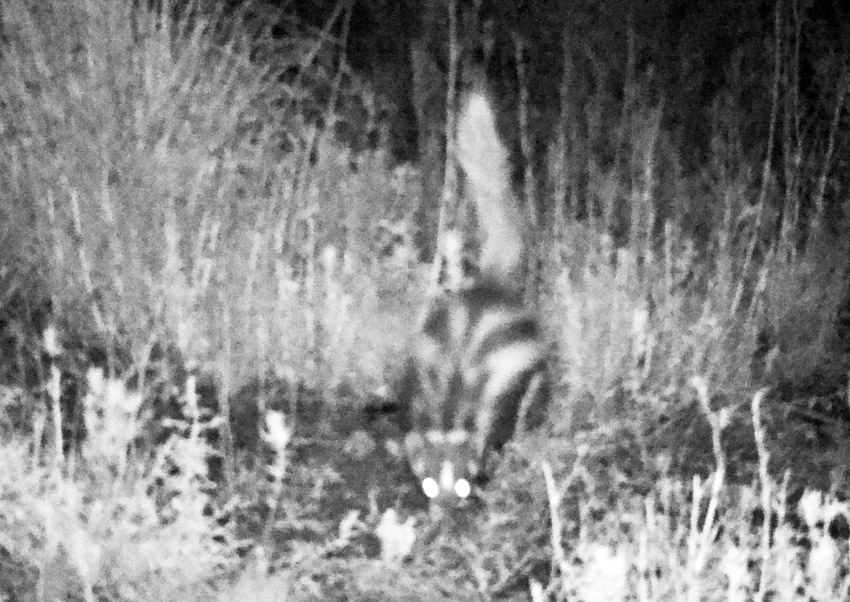A grainy black-and-white night vision photograph captures a skunk-like creature amidst a backdrop of tall grass and various foliage. The animal is positioned slightly off-center, and its large, reflective eyes stare directly at the camera. Its tail is arched upwards in an alert yet non-defensive stance, as if prepared to flee if necessary. The skunk's body displays a dark and bright striped pattern with noticeable white patches. The creature's back is arched, and its head is bent towards the ground, suggesting it could be foraging. All around, the scene is devoid of color, emphasizing the stark contrast of the nocturnal setting.